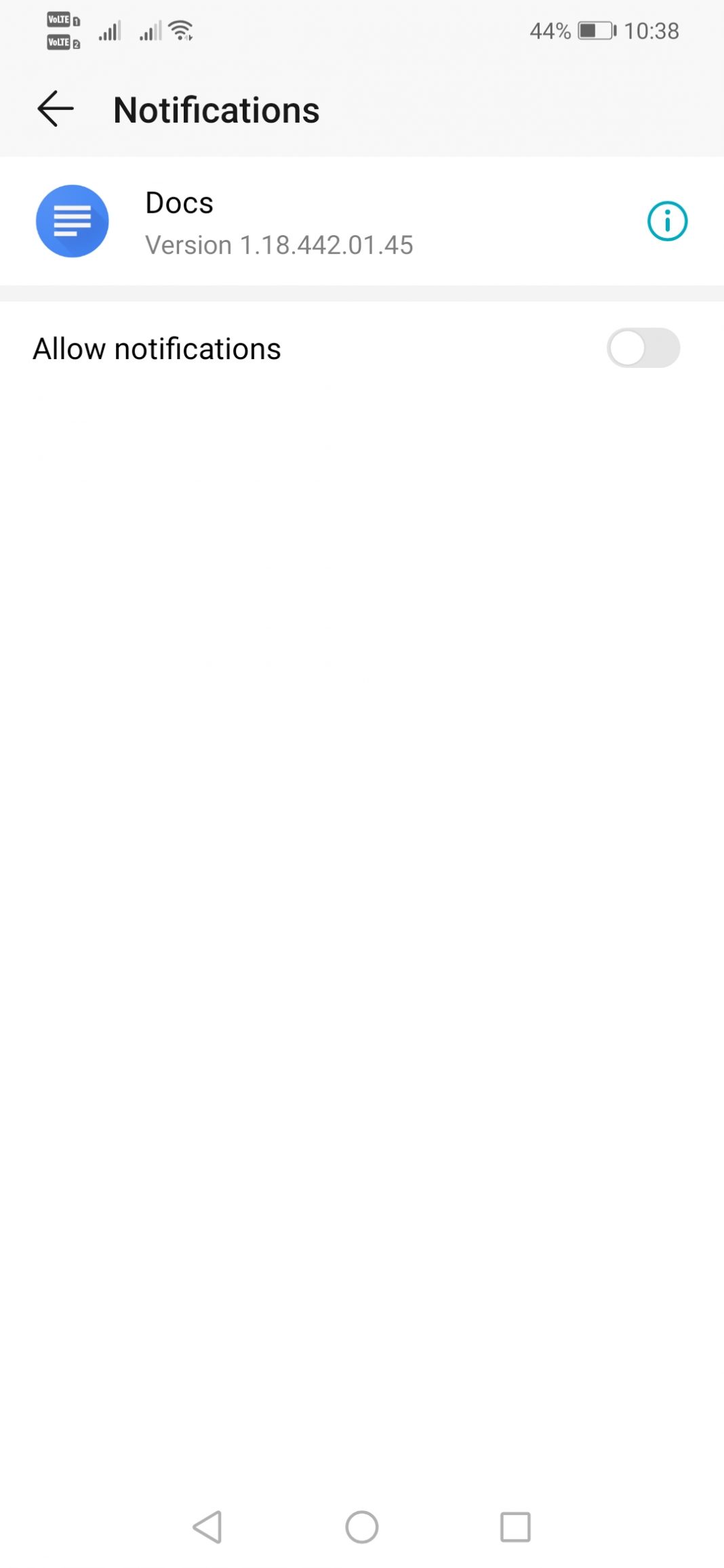In this image, we have a detailed screenshot of an Android device's display. The top left corner features dual network signal bars, both utilizing Voice over LTE technology. SIM 1 displays four out of five active bars, while SIM 2 shows three out of five bars. Adjacent to these indicators is the Wi-Fi signal icon, representing the device's current network connection.

On the top right of the screen, the battery icon reveals a charge level of 44%, and the time is precisely 10:38. Notifications are present, with one highlighting the DOCKS version, which is listed as 1.18.442.01.45, with a prompt reading “Allow notifications”.

At the very bottom of the screen, the familiar Android navigation keys are visible. These include the back button, the home button, and the recent apps button, arranged from left to right respectively. The screenshot captures a typical moment in the usage of an Android device, offering a clear view of its status indicators and navigation options.